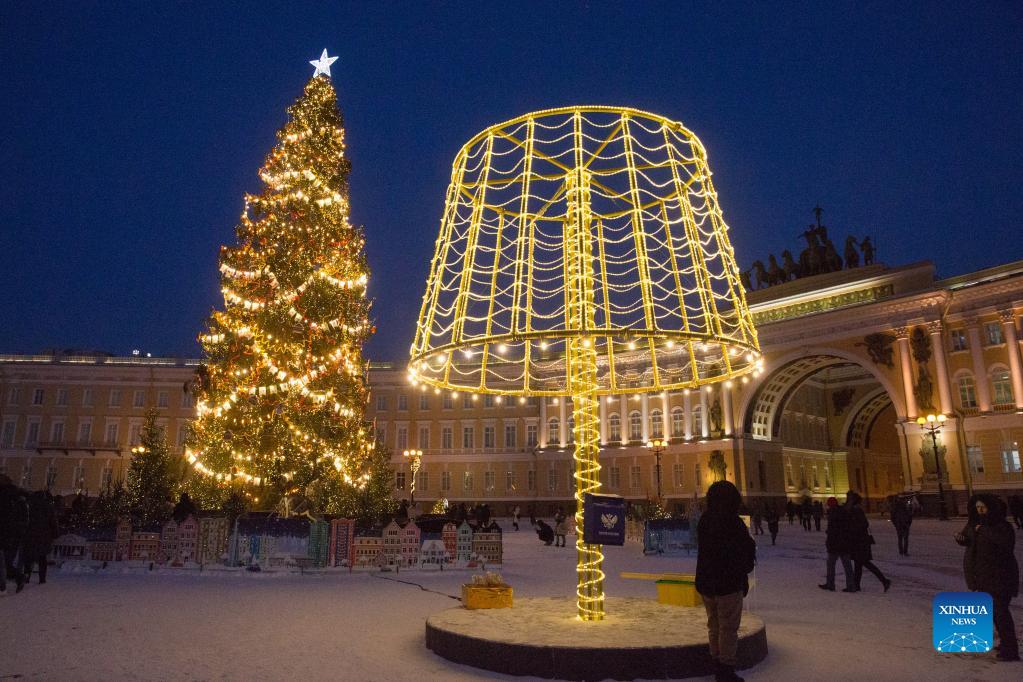The image captures a festive nighttime scene in what appears to be a European city. Dominating the foreground is a towering, 50-foot Christmas tree adorned with bright white lights cascading from its branches, topped by a prominent five-point star. Beneath the tree, a decorative setup features a model train and a small cityscape, adding an enchanting touch to the holiday display. Scattered around the tree are additional smaller, decorative Christmas trees.

The background showcases a colossal building wrapped around the plaza with multiple rooms and a grand arch entrance that looks walkable. Noteworthy is the decorative sculpture alongside the tree that resembles an illuminated lamp. The scene is set under a clear night sky, and the ground is blanketed with snow, heightening the festive atmosphere. Numerous people, many dressed in black, are seen strolling around, enjoying the display.

In the lower right corner of the image, a blue box with the text "Xinhua News" suggests that this photograph may have been sourced from a news site, possibly indicating an event of interest. The overall color palette of the scene includes shades of brown, yellow, white, and black, capturing the serene yet lively holiday spirit.